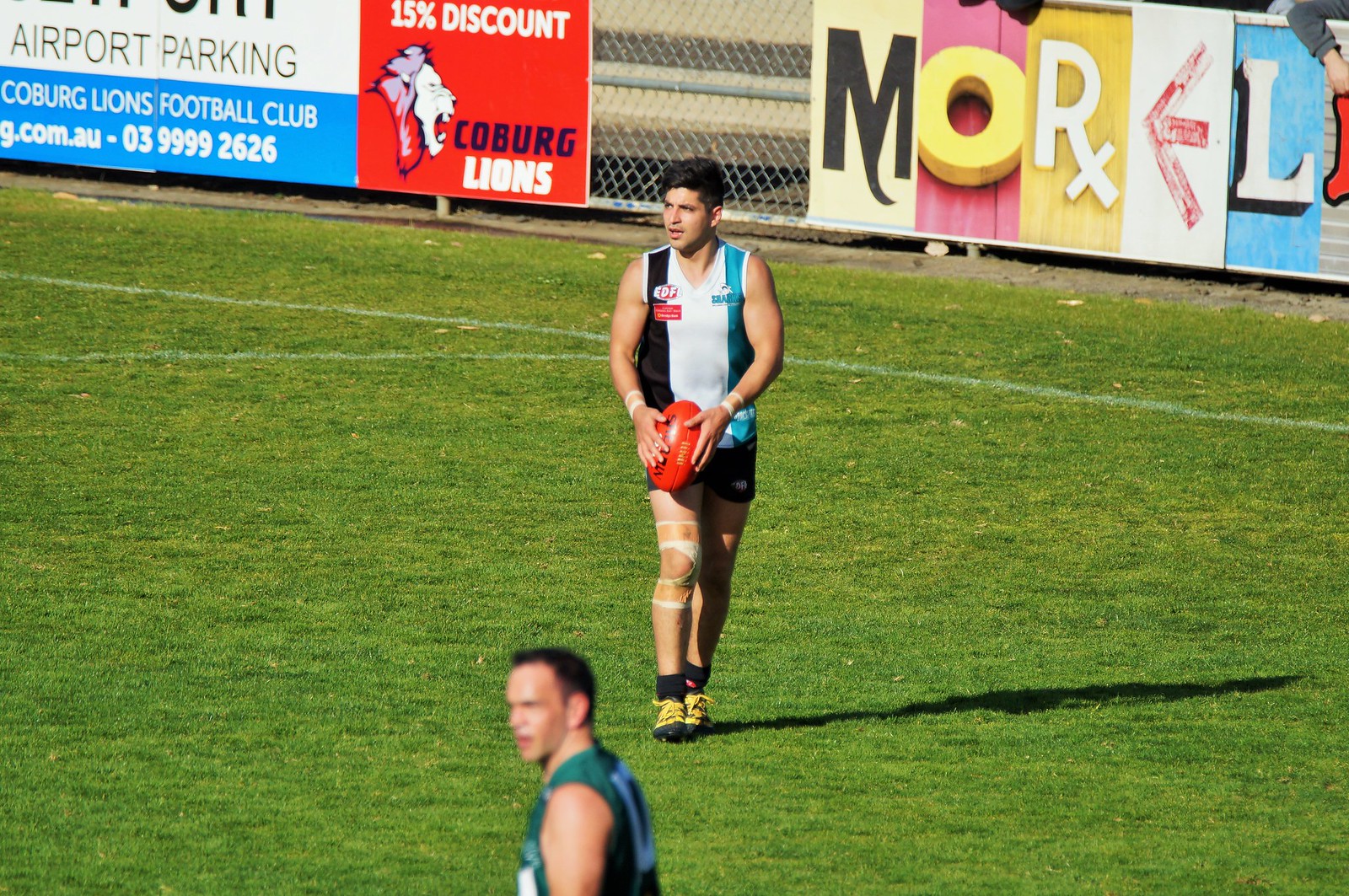An outdoor event captures a game on a grassy sports field, presumably rugby. Two men are the focal point, sporting casual athletic gear rather than traditional protective padding. The foreground features a white man with black hair, wearing a red, white, and blue tank top, black shorts, socks, and shoes, holding a large orange ball, likely indicating rugby. He has a brace on his right knee. Nearby, another man in a green tank top is partially visible. The perimeter of the field is lined with metal chain-link fencing adorned with billboards, advertising "Airport Parking Football Club, Coburg Lions 15% discount," and "More Rx." The scene includes hints that suggest an Australian context, such as references to "dot-com AAU" on one of the signs.